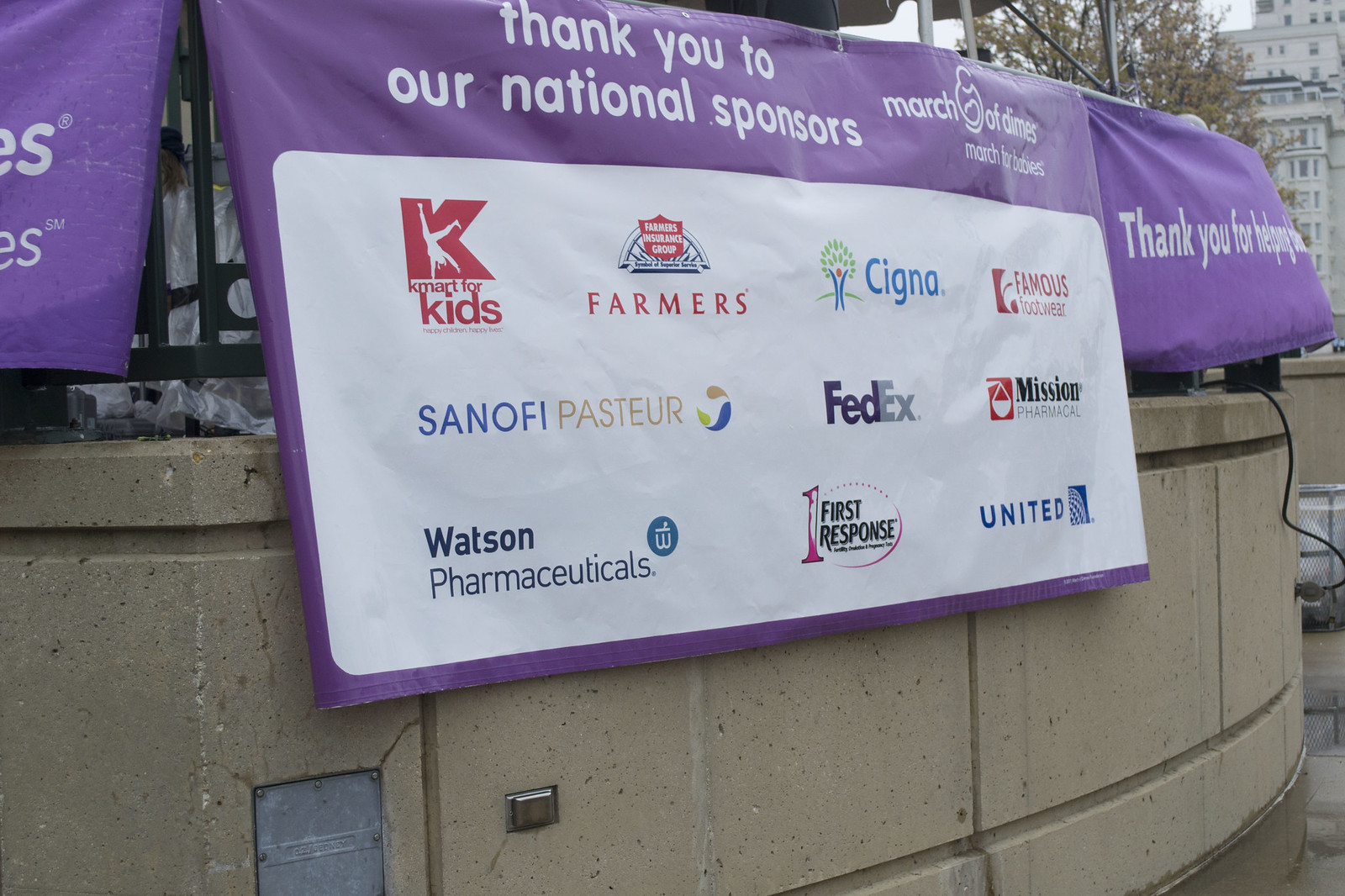In this outdoor daylight photograph, we see a curved platform or stage in what appears to be a park. The structure is made of poured concrete, and a green metal railing runs along its top edge. Draped over the railing are several purple banners. Prominently, the central purple banner features white text that reads, "Thank You to our National Sponsors," followed by logos of various companies such as Kmart for Kids, Farmers Insurance, Cigna, Famous Footwear, Sanofi Pasteur, FedEx, Mission Pharmaceuticals, Watson Pharmaceuticals, First Response, and United. This banner also includes the March of Dimes logo with the slogan "March for Babies." To the right of this central banner, another purple banner with white text reads, "Thank You for Helping." On the left side, only the letter 'S' is visible on another banner. In the background, the scene is framed by green leaves of trees and tall, light stone buildings, which are approximately 10 to 15 stories high.